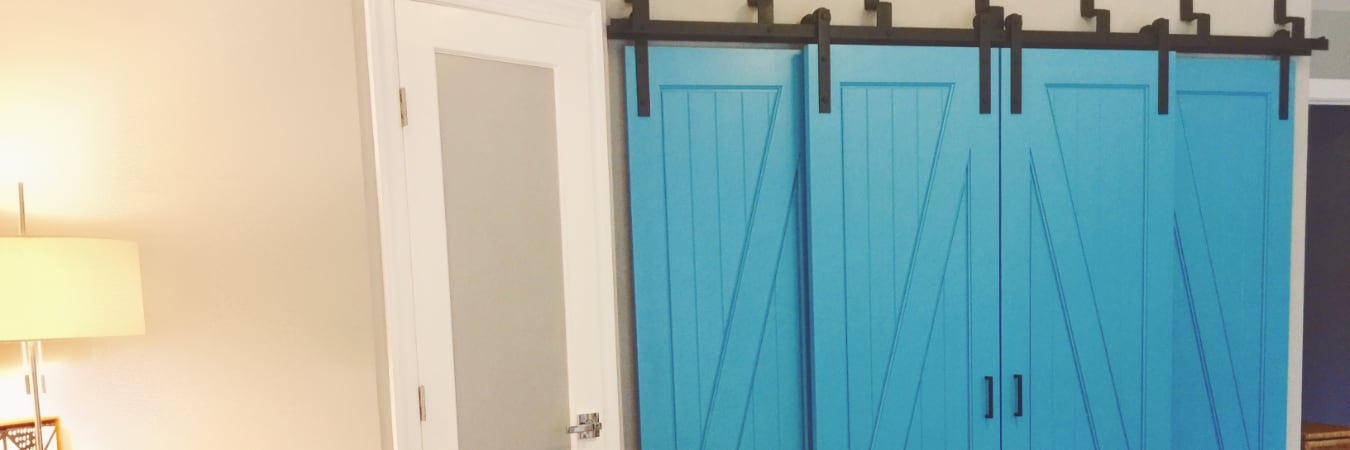In this detailed interior photograph, a harmonious arrangement of doors and lighting draws the eye. On the left side of the image, a cream-colored cylindrical lampshade is illuminated, possibly sitting on a piece of furniture against a white wall, with a hint of a photo frame beside it. Moving right, there is a distinct door featuring a white wooden frame with a frosted glass panel at its center. Dominating the scene just right of this door, a striking set of baby blue barn-style sliding doors, mounted on black metal rails, stretches horizontally. These wooden doors, composed of four intricately paneled sections, display a rustic charm with their diagonal plank design and black handles visible on two of the panels. Towards the far right, there’s an open doorway leading into a dimly lit adjacent room, creating a subtle contrast with the bright, detailed foreground. This well-organized composition captures the essence of a thoughtfully designed interior space.